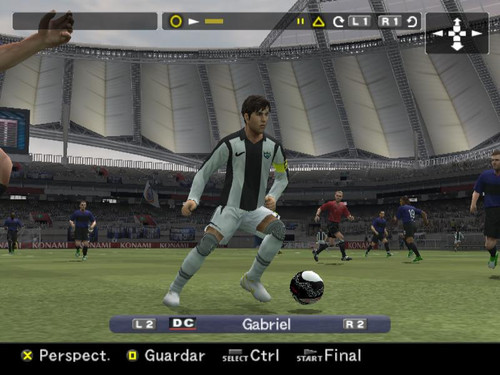The central image depicts a soccer player in mid-action, kicking a ball on a lush green field. Surrounding the player, at the bottom of the image, is a black-grey rectangular interface. On the left side of this interface, there is a grey section labeled "L2." Adjacent to it, a black segment features the letters "DC," followed by the name "Gabriel" and the notation "R2" on the right. Additionally, in the bottom-left corner, there is an "X" marked as "perspect." Continuing rightward, there are symbols including a square labeled "one R," a grey section with the word "select," a control button, and a start button labeled "final."

The upper part of the image showcases another black rectangle that includes icons representing a circle, a yellow and grey triangle, "L1," "R1," and a square indicating directional buttons pointing up, right, left, and down.

In the background, a wall or rooftop is visible, along with bleachers filled with enthusiastic fans. Centrally positioned is a soccer player in a uniform and cleats, actively kicking the ball. Surrounding this player on the field are various video game characters dressed in red, black, and blue uniforms, dynamically running in different positions across the field.